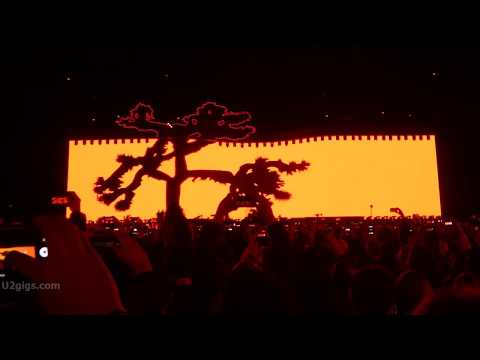In this photograph, we're presented with an intriguing night scene that features a large and engaged audience, presumably at a U2 concert held inside the innovative new stadium in Las Vegas. The image is steeped in a mix of red and orange hues, primarily due to the striking bright orange stage in the background, which appears to be an intricately designed screen resembling an upside-down notebook. The stadium's advanced 360-degree screen technology creates an illusion of an open sky, dotted with stars, adding to the surreal atmosphere. The crowd, comprising numerous individuals with their cell phones raised, is actively capturing the moment. The bottom left of the photograph includes a watermark, "U2Gigs.com," affirming the event's association with the renowned band. Additionally, amidst the orange backdrop, there appear to be dark shadows possibly depicting a large tree and some indistinct shapes, contributing to the mystical aura of the scene.